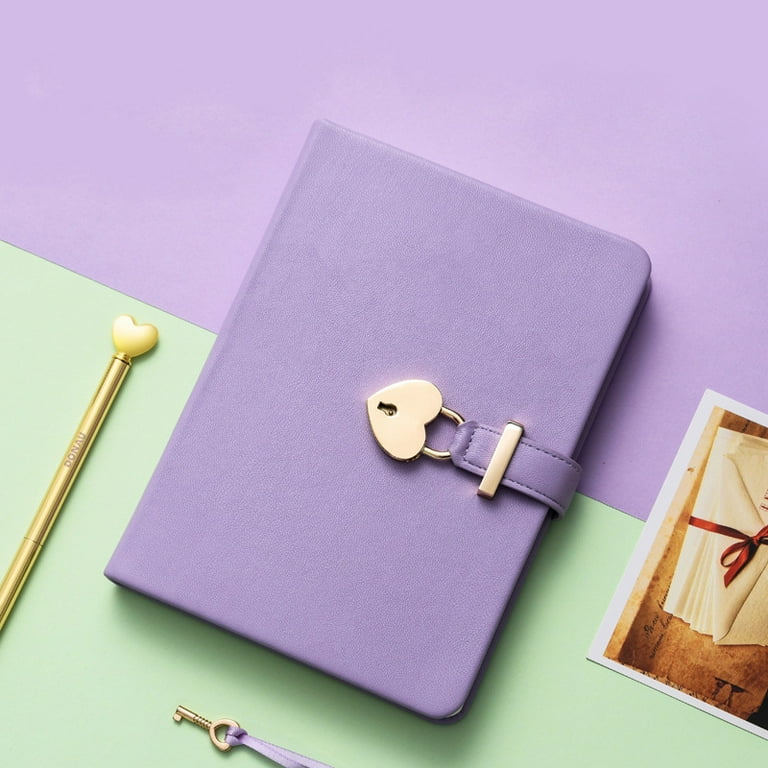The image depicts a detailed and vibrant scene set on a desktop divided equally between lavender and light green. The centerpiece is a purple-colored journal with a heart-shaped gold lock and a leather strap with a gold buckle. Accompanying the journal are several distinct items: a golden pen with a heart-shaped top, and a small gold skeleton key tied with a lavender ribbon. To the right, a Polaroid picture lies on the surface, showcasing a bundle of letters tied with a red ribbon. The meticulous arrangement and vivid colors create a rich and inviting composition.